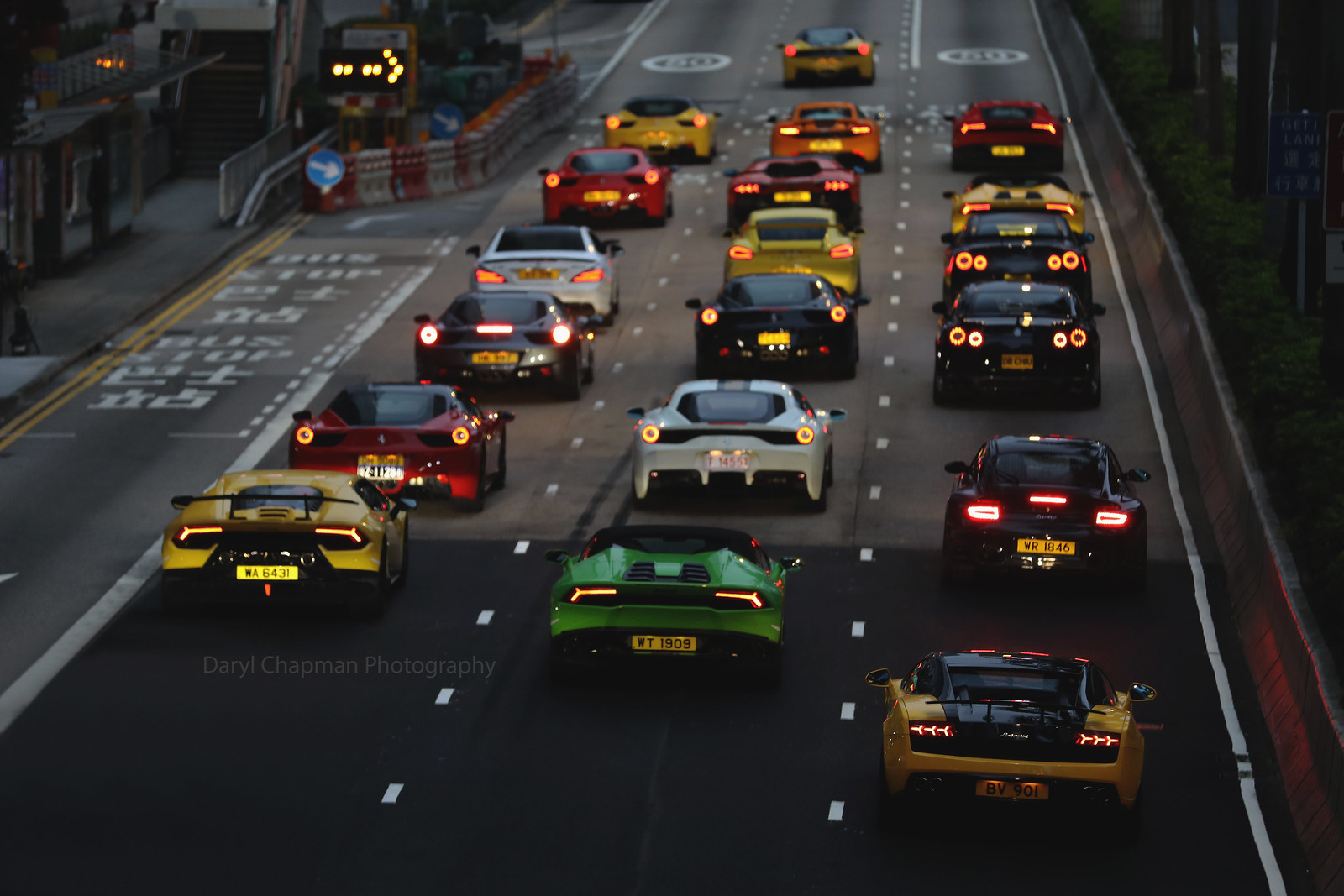The photograph captures a vibrant nighttime scene of a bustling urban street, possibly in Japan or another East Asian country, indicated by the Asian text on road markings and signs. The image features about 30 luxurious, modern sports cars in vivid colors like yellow, red, white, black, and a distinctive green car positioned centrally in the foreground. These cars are arranged in three lanes, with the addition of a fourth bus lane adjacent to a sidewalk lined with buildings. The brake lights of the cars cast a bright red and orange glow, emphasizing the dark evening setting as streetlights begin to illuminate. A lit traffic arrow is visible to the upper left, pointing to the right. This setting, captured with the watermark 'Daryl Chapman Photography,' distinctly highlights the opulent and futuristic design of the vehicles, complete with European-style license plates. The street features various road symbols including round markings, and wide white outlines and dotted lines, adding to the organized yet dynamic urban atmosphere.